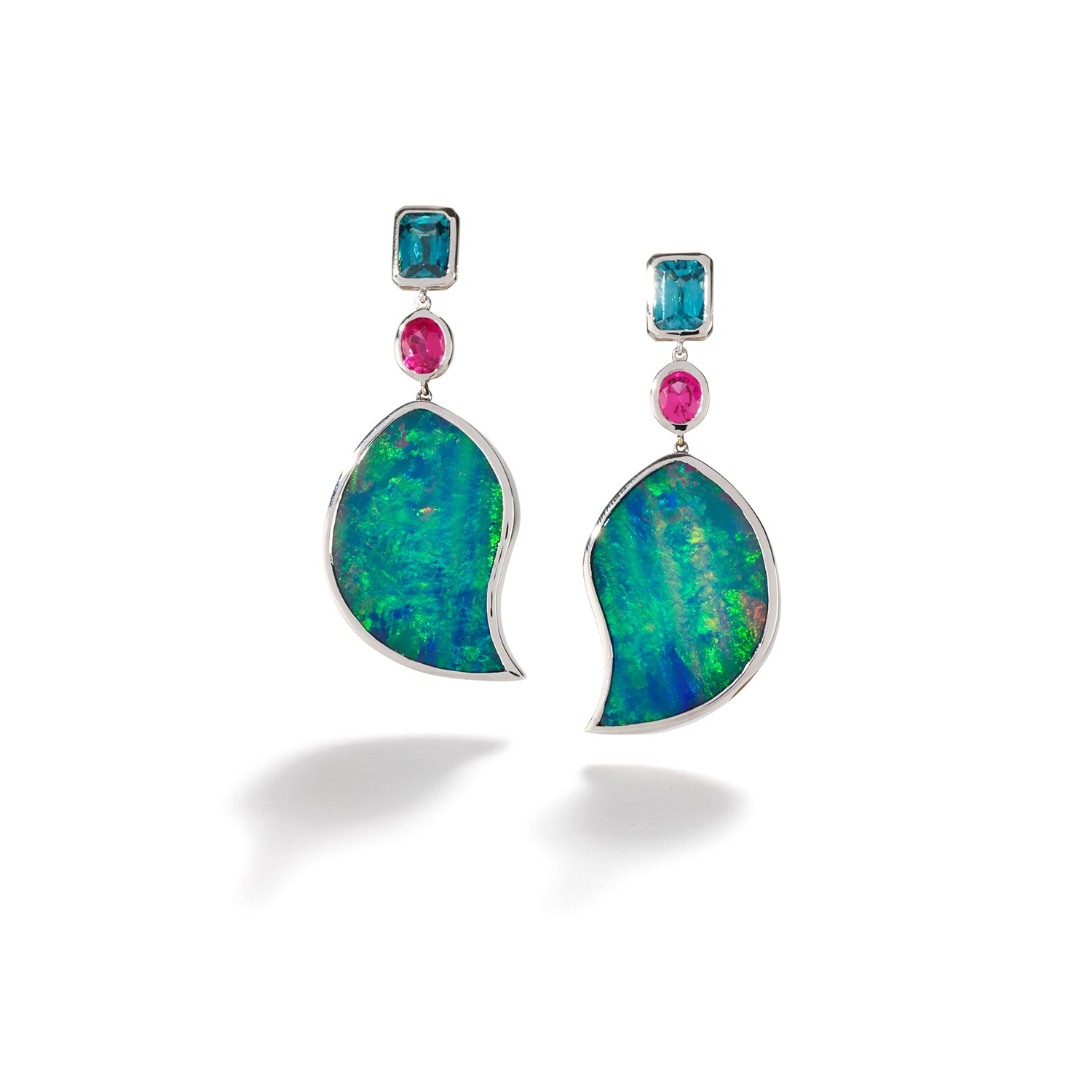This image features a pair of intricately designed, dangly earrings displayed against a white background. Each earring consists of three distinct segments, all exquisitely outlined in silver or platinum.

The top segment of the earrings is a vertically oriented, elongated square, each housing a medium blue gemstone adorned with a series of darker, horizontal and vertical lines. This section resembles a light blue sapphire or opal, providing a striking start to the piece.

Dangling from the blue gemstone is an oval-shaped, bright pink stone, adding a vibrant splash of color. This pink gem acts as the midsection and is seamlessly connected to the more complex, bottom segment.

The bottom segment is an elongated teardrop or leaf-like shape, also bordered in silver. Its backdrop is predominantly blue but is richly interspersed with splashes of green, suggesting an earthy, agate-like appearance. There may be subtle hints of yellow and orange within this segment, evoking an artistic representation of the Earth with its varied tones and hues.

Notably, the earrings are designed to complement each other asymmetrically; the left earring sits slightly higher than the right, creating an illusion of harmony and balance, much like complementary puzzle pieces. They appear to be hanging freely, further highlighting their delicate craftsmanship and stunning design.